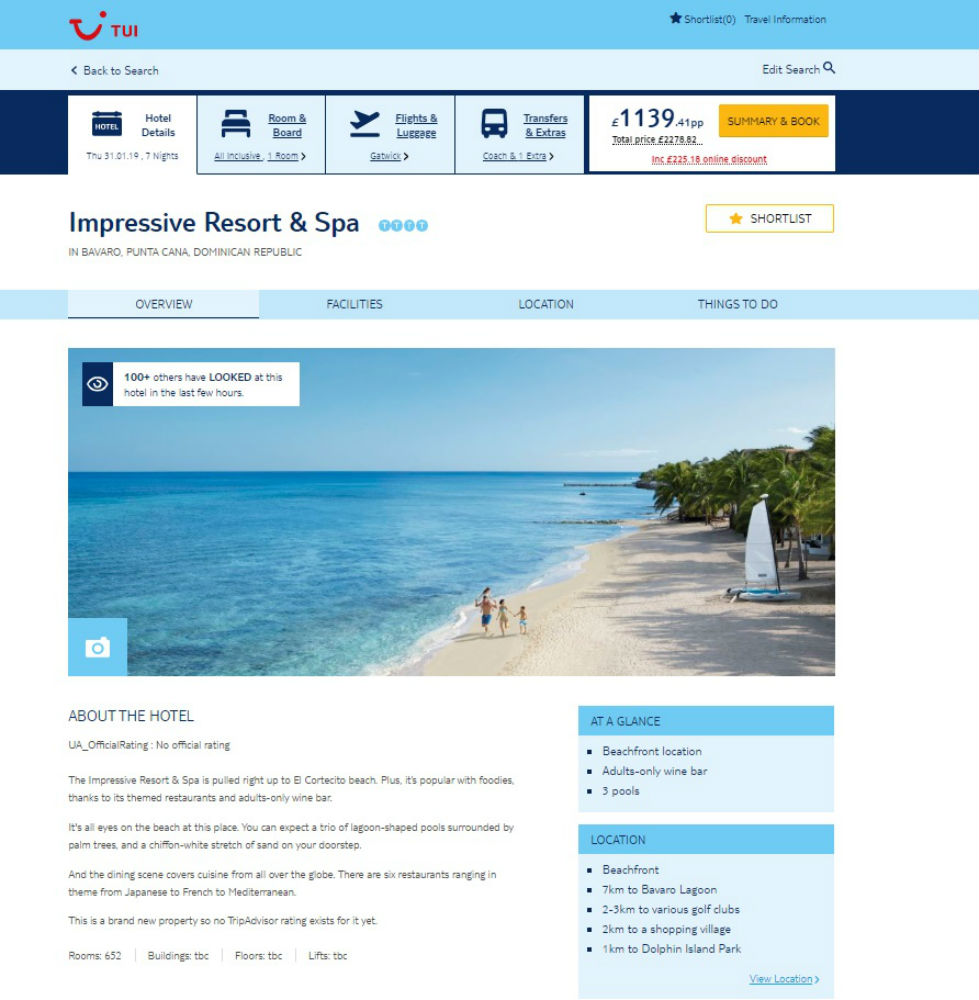**Impressive Resort and Spa Overview - Bavaro, Punta Cana**

At the top of the resort's webpage, a light blue bar spans from left to right, featuring the bold red letters "TUI" alongside a distinctive logo that resembles a face with one eye and a mouth. This bar offers options to return to or edit your search. 

Immediately below, the navigation menu includes links to hotel details, room and board, flight, luggage, transfers, and extras. The main content begins with the headline: "Impressive Resort and Spa in Bavaro, Punta Cana, Dominican Republic."

The page provides various sections: Overview, Facilities, Location, and Things to Do, with the Overview tab currently selected. 

A captivating image dominates the page, showcasing an idyllic beach scene. The ocean's crystal-clear waters meet an almost-white sandy shoreline. A family—comprising a father, mother, and two children—enjoys the serene setting. Palm trees frame the right side of the image, with the ocean to the left and clear skies above. In the distance, a small sailboat, possibly a catamaran, is visible on the water.

The hotel's description below the image states that the Impressive Resort and Spa is located right on El Cortesito Beach. It's particularly favored by food enthusiasts, thanks to its themed restaurants and adults-only wine bar. The beachfront location features lush landscapes including a trio of lagoon-shaped pools surrounded by palm trees and a long, white sandy beach right at your doorstep. The dining facilities at the resort offer a global culinary journey with six themed restaurants showcasing Japanese, French, and Mediterranean cuisines, among others. As a brand new property, the resort currently doesn't have a TripAdvisor rating. 

This detailed presentation emphasizes the resort’s luxurious amenities, scenic beauty, and gastronomic delights, making it a highly appealing destination for potential visitors.